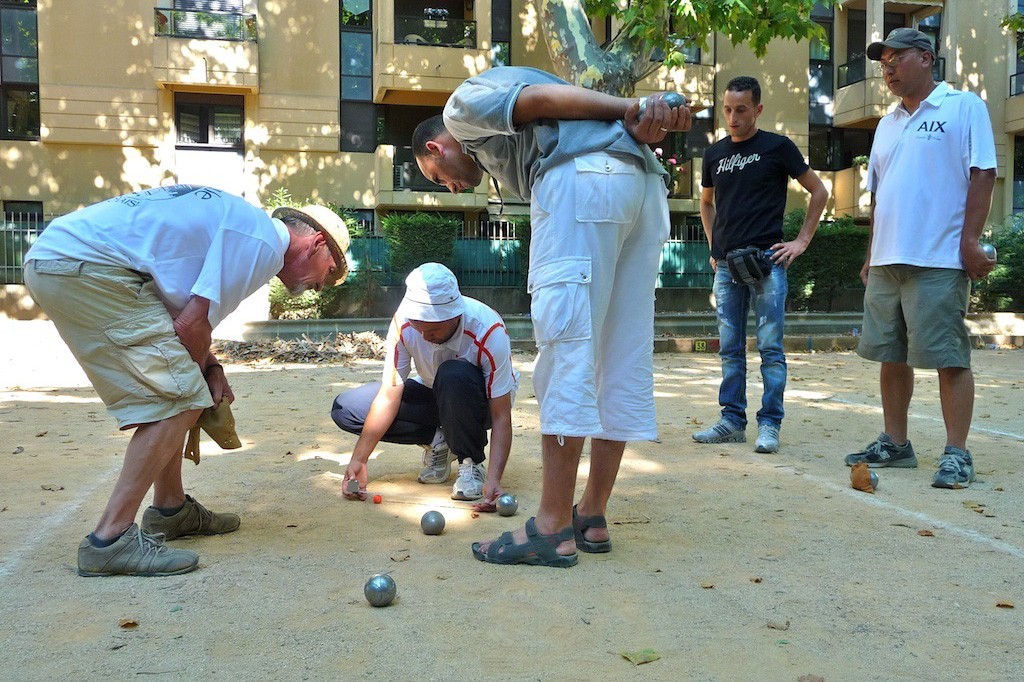Four adults are absorbed in a spirited game of marbles in a sandy area marked with chalk lines. Their attire varies; one sports a pair of white capris, another wears blue shorts paired with a white polo shirt bearing the logo "AIX," while the third player is clad in navy blue slacks. The final participant is dressed in jeans and a black t-shirt with "Hill Figure" emblazoned in white across the front. The marbles they are using are noticeably large. The player in the white capris is intently bent at a 90-degree angle, closely inspecting the marbles on the ground. They are playing in front of a yellow building that appears to be a housing complex. A green fence, partially covered with creeping plants, stands behind them, along with a tree that adds a touch of greenery to the scene.